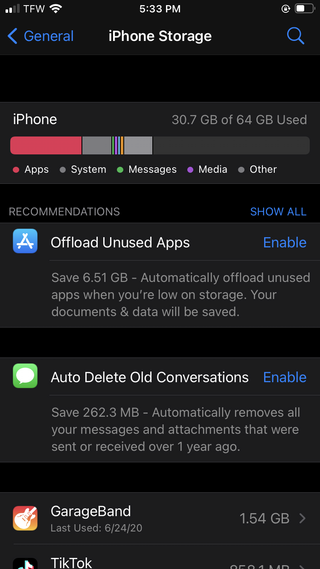This screenshot is a vertical image captured from an iPhone, displaying the 'iPhone Storage' settings. The background is a solid black with a slight gradient to a lighter black at the top for the status bar.

At the top left corner, the signal strength indicator, labeled 'TFW', is visible alongside the Wi-Fi symbol. Centered at the top is the current time, displayed as '5:33 PM' in white. To the right, the status icons include a circular arrow and a battery life indicator.

Underneath the status bar, an arrow pointing left appears in the upper left corner, with 'General' labeled in blue text next to it. The middle of this section reads 'iPhone Storage' in white. On the upper right side, there's a blue magnifying glass icon.

Below this, a gray rectangle shows a bar graph illustrating storage usage. The bar is color-coded: red (for apps), gray, and several other colors depicting different categories, followed by more gray. It indicates '30.7 GB of 64 GB used.' Beneath the bar, categories such as apps, system, messages, media, and other are listed with their corresponding colors.

The section below provides storage recommendations, including options to 'Offload Unused Apps' and 'Auto Delete Old Conversations,' both of which can be enabled. 

At the bottom of the image, available apps are listed by storage usage. 'GarageBand' uses 1.4 GB, while 'TikTok' is partially visible, indicating additional details are cut off.